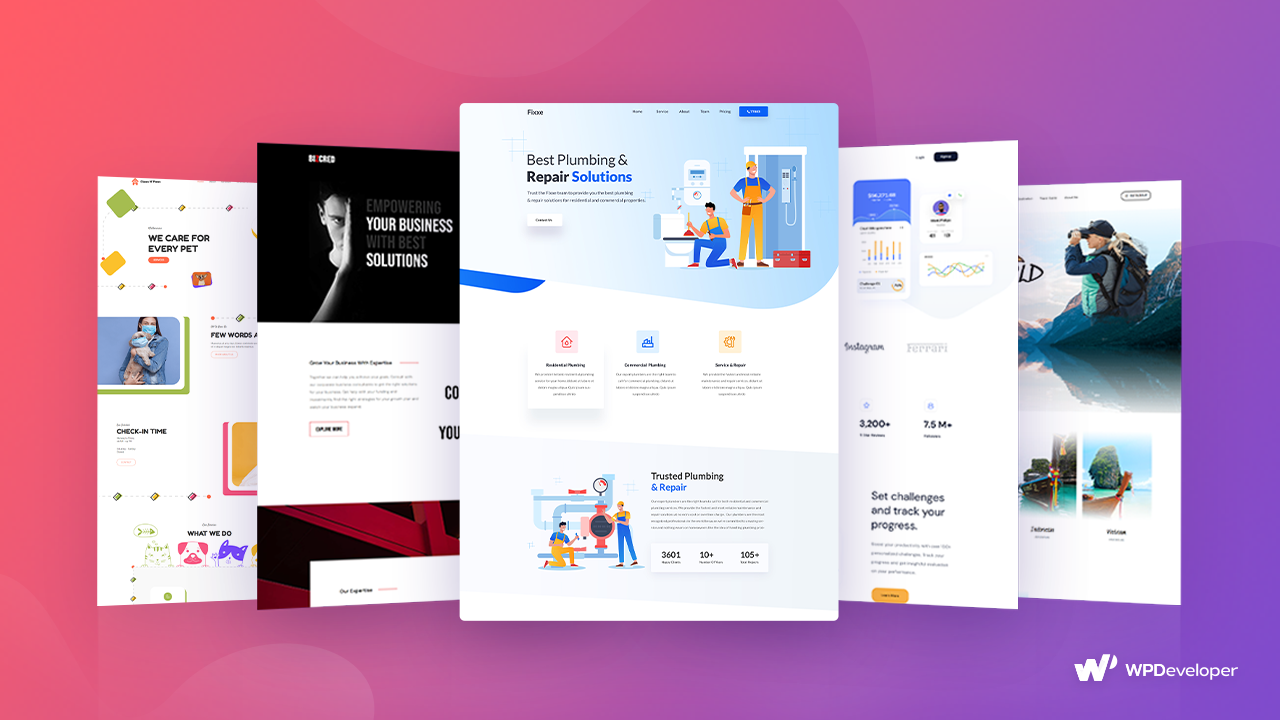The image is a horizontal rectangle with a gradient background transitioning from pink on the left to purple on the right. At the center of the image, there are six distinct pieces that resemble printed web pages or developer mock-ups. In the bottom right corner, there's a letter "W" accompanied by the phrase "WP Developer."

Among the various pages, the central one stands out with its blue and white design—blue on the top and white on the bottom. It features text reading "Best Plumbing and Repair Solutions," along with an illustration of a bathroom. In the illustration, one person is kneeling and using a plunger on a toilet, while another individual in yellow overalls stands nearby. There’s also a toolbox to the right of them. The lower section of this page includes another heading: "Trusted Plumbing and Repair," with more plumber illustrations.

Additionally, one of the other pages has a black top and showcases an image of a man with a hand partially covering his face, coupled with the text "Your Business Solutions." There’s more text on the page, though it is not entirely legible.

Overall, the image appears to be showcasing web development templates or examples associated with a website developer, likely specializing in WordPress given the "WP Developer" label.